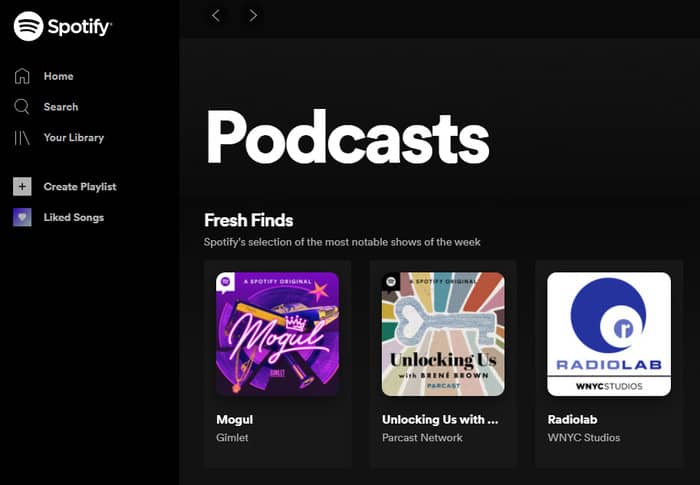This image depicts a Spotify interface designed with a sleek, black background. In the upper left-hand corner, the Spotify logo is prominently displayed. Below it, a round icon with dynamic, curved red and black lines is featured. On the left sidebar, there are tabs labeled "Home," "Search," "Your Library," "Create Playlist," and "Liked Songs," each accompanied by corresponding icons. 

Dominating the central part of the interface, the word "Podcasts" is boldly written in large white text. Beneath this heading, "Fresh Finds" is introduced with a smaller subtitle that reads, "Spotify's selection of the most notable shows of the week." 

Showcased below are three podcast thumbnails. The first podcast, "Mogul," is set against a purple background with a star icon and stylish script, showcasing "Mogul Gimlet" underneath. The second podcast, "Unlocking Us," features a palette of green and brown and mentions its association with Paracast Network. The third podcast, "Radio Lab," is illustrated with a white box that contains the podcast's title along with the banner "WNYC Studios," accompanied by a blue circle containing smaller concentric circles.